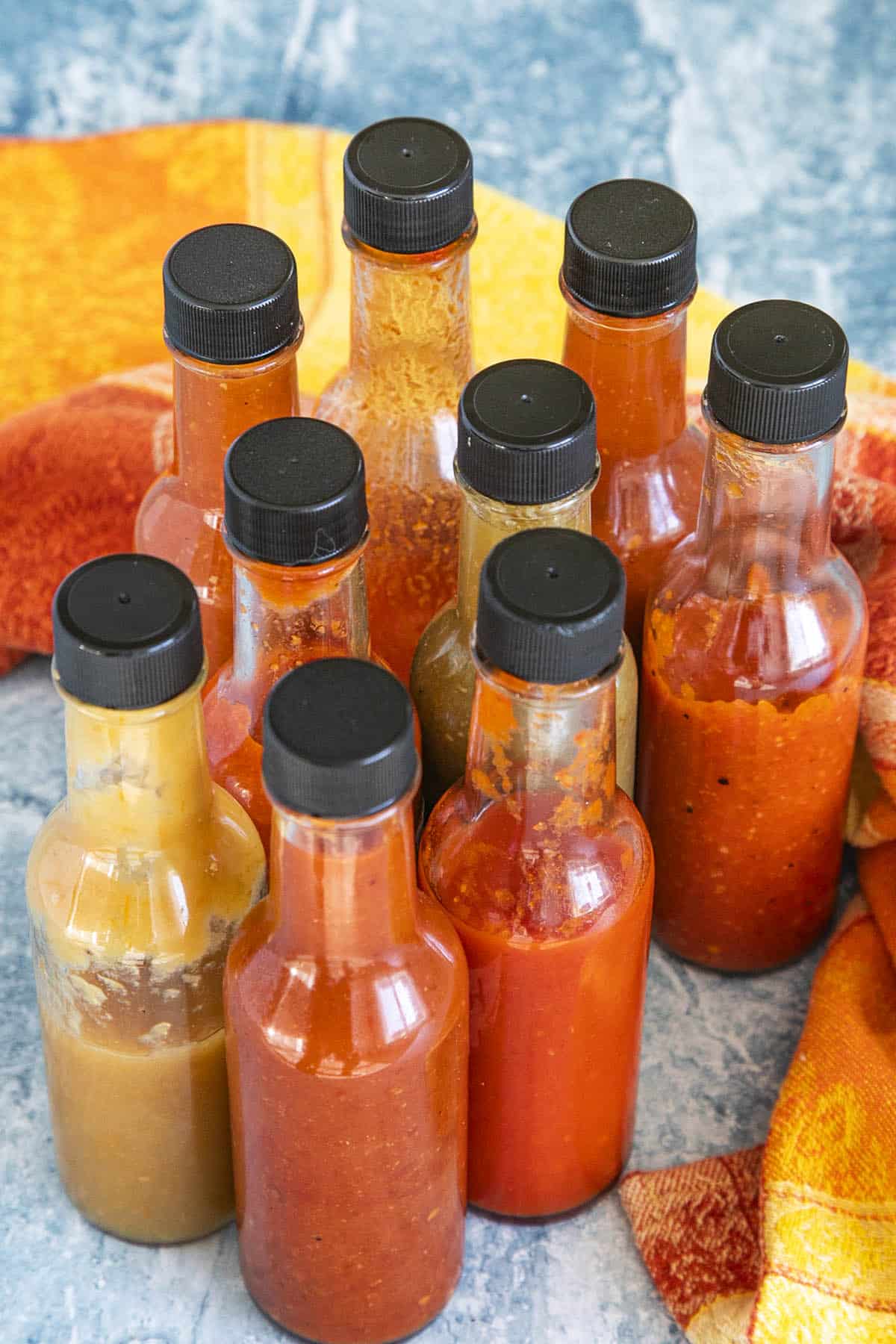The image depicts nine assorted bottles of sauces, prominently featuring hues of deep red, bright orange, and green. Among the bottles, some have full contents while others appear partially used, showing remnants of sauce in their necks. The sauces tend to be dense, with one solid red bottle and another featuring speckles, suggesting different varieties. The bottles are arranged upright on a blue-gray countertop with a marble-like pattern. A vibrant, floral-patterned dish towel with shades of terracotta, bright orange, and yellow is visible behind the bottles and to the right. The various colors and used states of the bottles give the impression of frequent use in a lively kitchen setting.